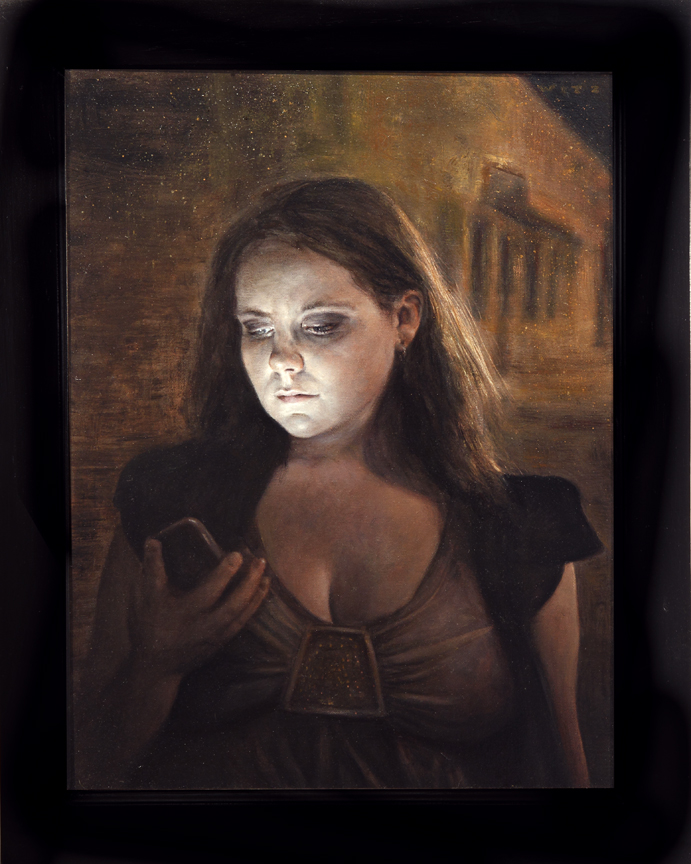The image is a lifelike painting depicting a young, fair-skinned woman with long brown hair. She is holding a cell phone in her right hand, her arm bent at the elbow, and she is looking intently at the screen. The phone's whitish glow casts an eerie light on her face, highlighting her dark eye makeup, which gives her a tired and serious expression. Her hair, slightly wispy, frames her face. She is dressed in a revealing low-cut blouse with flowy, bunchy lines and a prominent buckle or decorative element in the center of her chest. Over this, she wears a black cardigan or shoulder design, which adds contrast to her attire. In the background, there is a dark brownish-orangish building with yellow tones, which appears to converge to a point, adding depth to the scene. The details in the painting masterfully blend realism with an emotional undertone, creating a striking and somewhat unsettling visual.